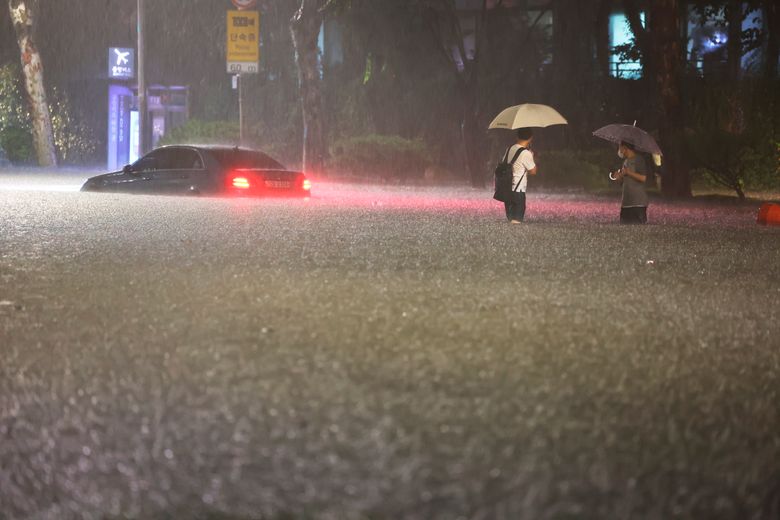The photograph captures a surreal nighttime scene of a flooded street, still being drenched by heavy rain. In the foreground, a four-door passenger car is stopped, with its brake lights casting an eerie red glow across the gray-green water, which is almost as high as the top of the tires. Rain continues to fall heavily, creating splatters on the surface of the standing water, which reflects pink and red hues from the car's lights. 

To the right of the car stand two men facing each other. The first man, closer to the camera, has his back to us, wearing a white t-shirt, dark shorts, and a black backpack. His cream-colored umbrella shields him from the downpour, and the water reaches up to his thighs. The second man, positioned in front and turned slightly away, sports a gray t-shirt, dark shorts, and a gray umbrella. The water is nearly crotch-deep for him. Both men appear to be of Asian descent, with dark hair and face masks, emphasizing the ongoing rain and flood.

In the background, a blue airport sign featuring an airplane icon and the number '60' stands in contrast to an orange and black sign, indicating a possible bus terminal. The scene is framed on the right by dense woods and trees, adding to the ominous atmosphere of the flooded street.